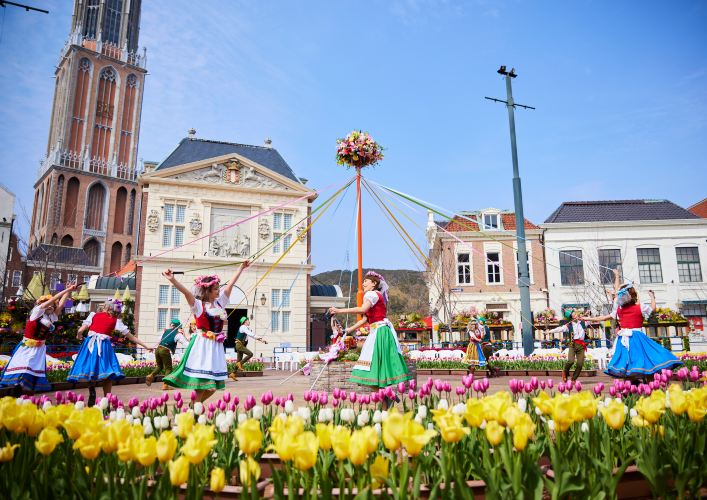The image captures a vibrant Maypole celebration, possibly set in a European country like Holland, Switzerland, or Sweden. At the center of the scene is an orange pole adorned with a bouquet of flowers at the top. This focal point is encircled by about ten ropes, each held by a participant dressed in colorful attire. The dancers, both men and women, form a lively circle around the pole, moving either clockwise or counterclockwise. The men are dressed in olive green pants, light brown shoes, and green hats, while the women are adorned in light blue and green skirts, white aprons, and flower crowns.

Tulips in hues of yellow, pink, white, and red decorate the foreground, enhancing the festive atmosphere. The celebration seems to take place in a plaza or roundabout, surrounded by various European-style buildings. To the left is a tall, brown, stacked building with a progressively narrower structure. Adjacent to it stands an ornate white building with multiple stories. Further right is a two-story brown residential building and a white office building with a black roof. In the background, there are fields or empty spaces, framed by additional buildings including a tan one with a red roof and white dormer.

Overall, the photograph depicts a joyful and traditional celebration, rich with cultural and architectural details.